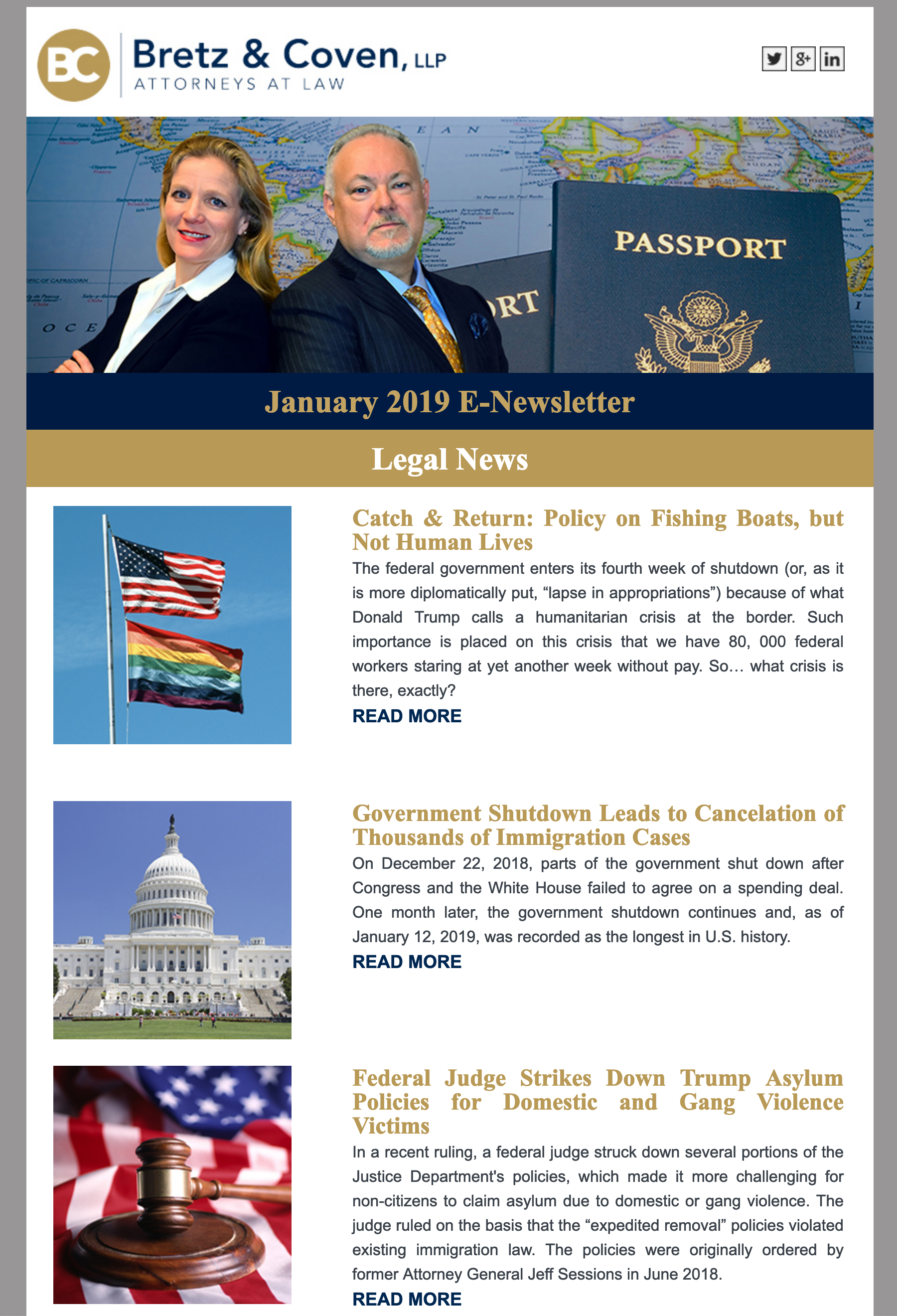**Screenshot Description: Bretts & Coven, LLP January 2019 E-Newsletter**

In this screenshot of an online newsletter from the law firm Bretts & Coven, LLP, the title of the firm is prominently displayed in the top left corner. Directly below the firm's name is a small social media button, adjoining a banner photo that showcases a professional woman in a suit with arms crossed, standing back-to-back with a suited man. The backdrop of this banner features a world map and large images of passports, suggesting the firm's specialization in immigration or international law.

The newsletter's header reads "January 2019 E-Newsletter," followed by a section titled "Legal News." This edition highlights three articles:

1. **"Catch and Return: Policy on Fishing Boats, Not Human Lives"**
   - Preview: A brief overview of the article's focus.
   - Read More button for full access.

2. **"Government Shutdown Leads to Cancellation of Thousands of Immigrant Cases"**
   - Preview: A summary of the article's content.
   - Read More button for full access.

3. **"Federal Judge Strikes Down Trump Asylum Policies for Domestic and Gang Violence Victims"**
   - Preview: A snippet of the article's details.
   - Read More button for full access.

This neatly structured e-newsletter offers detailed insights into current legal issues related to immigration, underscoring the expertise of Bretts & Coven, LLP in this specialized field.